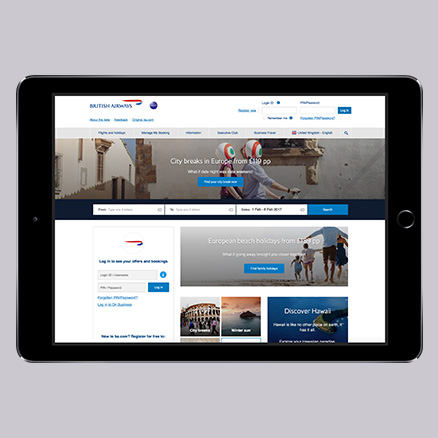This image captures a screenshot of an iPad displaying the British Airways website in landscape orientation. The iPad, with a black border, rests on a gray background. The top section of the website features a prominent British Airways logo positioned on the left side of a large header. The header's menu appears somewhat disjointed, with five or six floating options on the right, whose placement seems a bit unclear. 

Beneath the header is a grey bar containing a more traditional navigation menu with approximately six or seven options. The main highlight of the webpage shows a hero image depicting two individuals riding a motorcycle in what appears to be a European setting. They are wearing mostly white helmets adorned with target designs featuring red circles and green dots. The background showcases an old white building, enhancing the European ambiance. 

A text overlay on the hero image promotes "City Breaks in Europe from..." though the specific price is not legible. Below this are search fields likely for entering destinations (to and from) and travel dates. Further down, the page displays various travel destination thumbnails, including people frolicking on a beach, a glimpse of the Colosseum in Rome, an island paradise, and an invitation to "Discover Hawaii," among other travel-themed visuals. Search options are also available on the left side of these images, reinforcing the typical layout of a travel website.